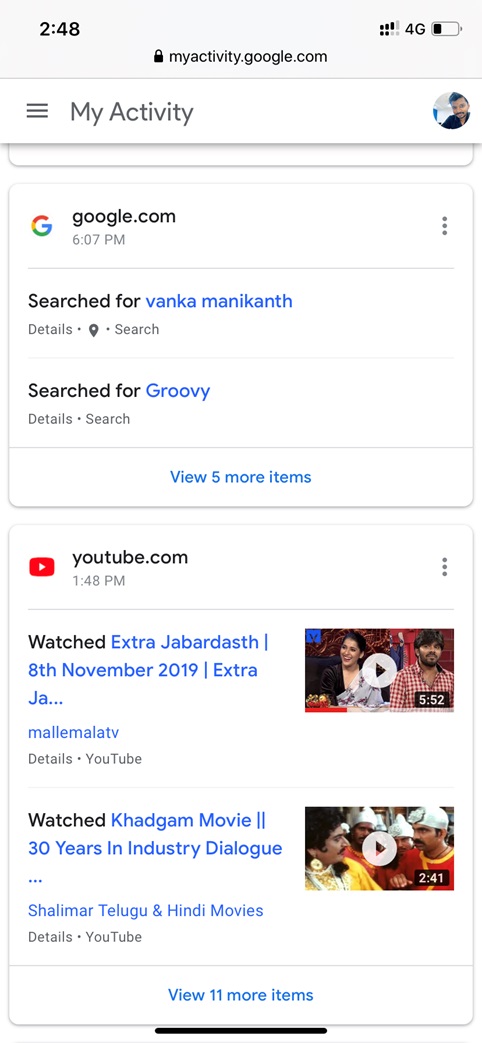The image showcases the screen of a cell phone displaying the "My Activity" page on Google. At the top center, the URL "myactivity.google.com" is visible, confirming the page being viewed. The time shown on the phone's interface is 2:48 PM, located at the upper left-hand corner. The phone operates on a 4G network, also indicated at the top. The battery icon on the upper right is displayed horizontally and appears to be about one-third full with a black section indicating the remaining charge.

Below this, the page features a profile picture of a man with dark hair, slightly dark skin, a mustache, and a beard. The page is predominantly white with blue clickable links and segmented sections for different activity items recorded by Google.

The first recorded activity shows that at 6:07 PM, the user searched for "Venka Manekantha" on google.com. Additional options under this entry include "Details" and "Search." This is followed by another search for "Groovy" and a note to "View five more items," indicating additional activity not fully displayed.

Further down, at 1:48 PM, an entry from youtube.com notes that the user watched a video titled "Extra Jabberdash," with the date marked as November 8, 2019. The truncated note "Extra JA..." likely signifies "Extra Jabberdash," and the attribution goes to "Malamala TV."

Towards the bottom, more sections suggest additional recorded activities, with a prompt to "View 11 more items," implying several other interactions that can be expanded to view in detail.

The page is structured to provide a comprehensive log of the user’s recent activities, sorted by service and timestamp.